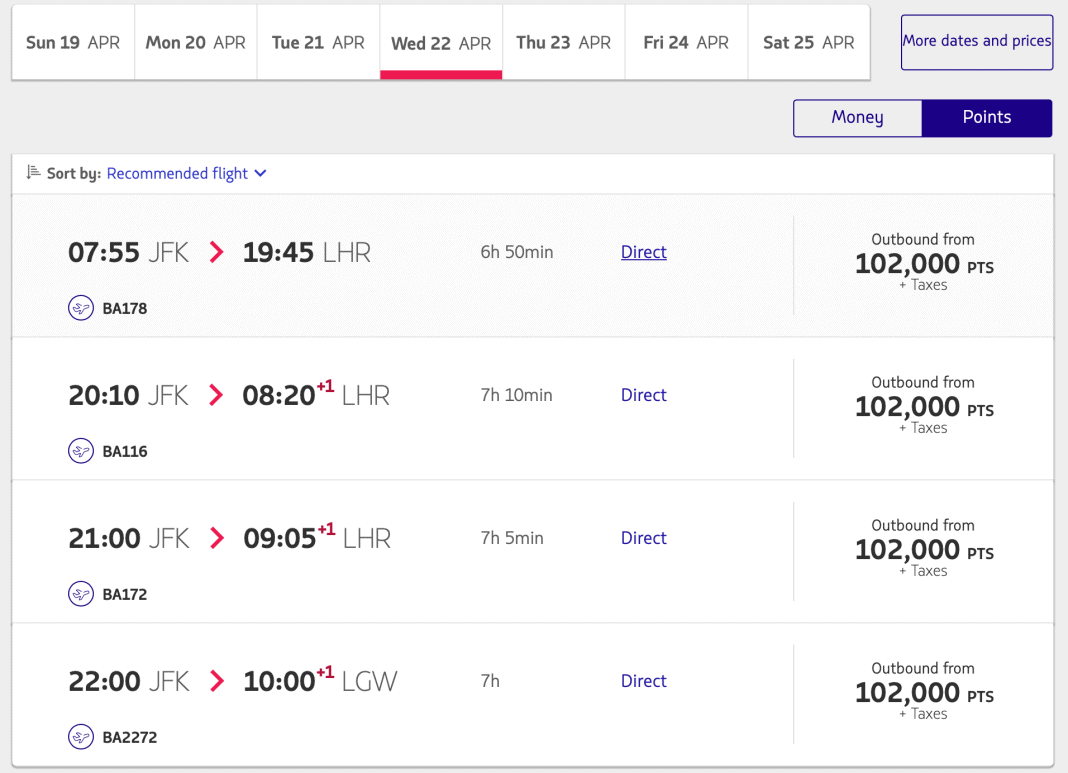The image depicts a flight booking website with a minimalist design characterized by a gray background and alternating white and lighter gray tables, featuring black text for optimal readability. The primary accent colors used throughout the website are purple and red.

At the top of the page, there is a navigation table displaying various dates: Sunday, 19th April; Monday, 20th April; Tuesday, 21st April; and the currently selected Wednesday, 22nd April, which is emphasized with a bold red underline. Further dates are shown as Thursday, 23rd April; Friday, 24th April; and Saturday, 25th April. A "More Dates and Prices" button is also present, presumably offering additional options and information.

Nearby are filter options labeled "Money" and "Points," with "Points" currently selected. This selection is visually indicated by a purple background with gray text, while the other options are shown with a gray background and purple text.

Below the date selection, there's a sorting option with a dropdown menu currently set to "Recommended Flights." This is followed by a listing of various flights departing from JFK to either LHR or LGW, all of which are six to seven hours long. Each listing mentions whether the flight is direct, highlighted in purple text.

On the far right, there is a summary of the outbound flight details and a column displaying prices in points, inclusive of taxes.